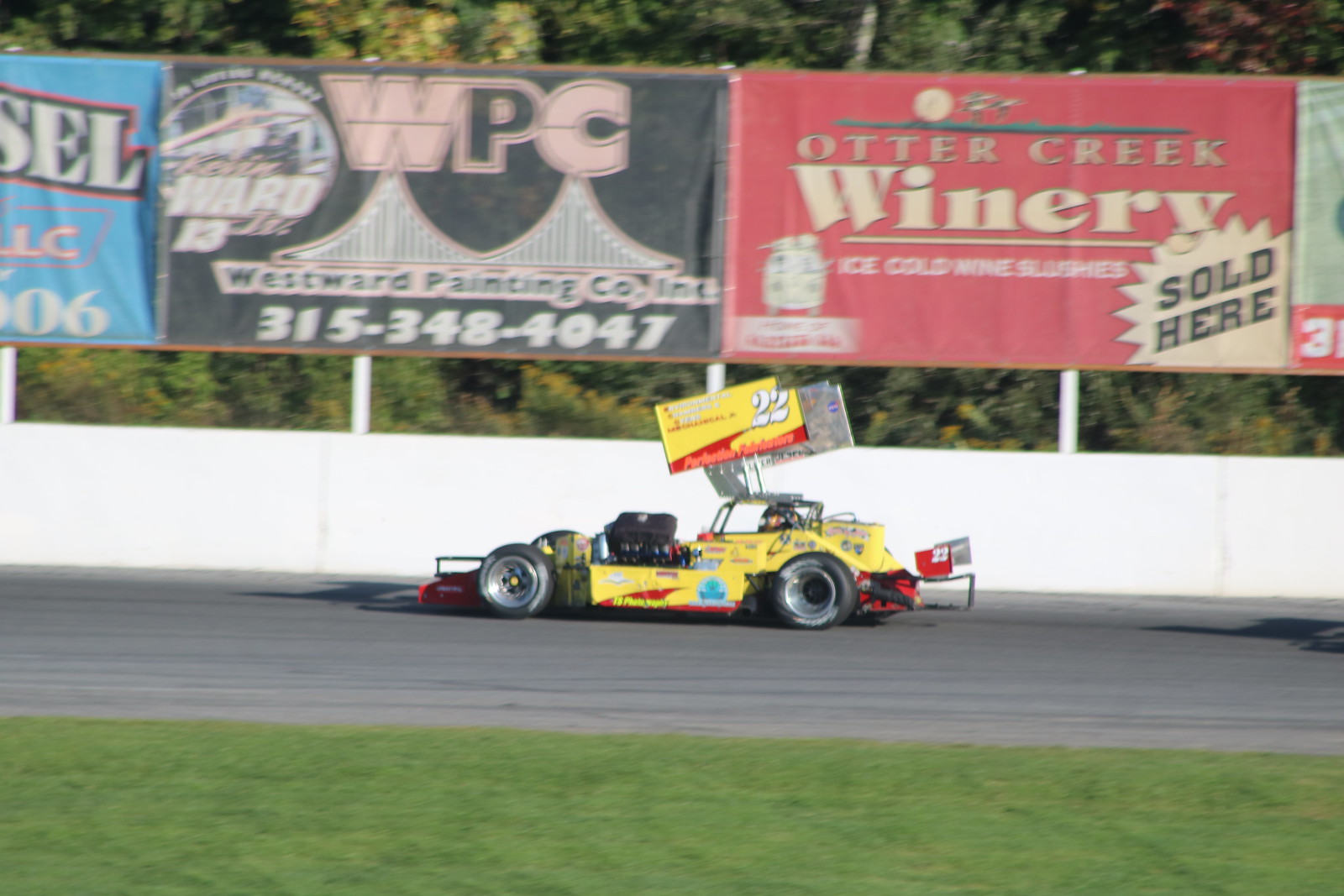The image captures a vibrant scene at an auto racing show, featuring a meticulously crafted race car on a gray road. The car appears to be an F1 model, predominantly showcasing bright yellow and red colors, with a hint of light blue and various sponsor logos that are not clearly visible. It bears the number "22" prominently displayed on the upper section and tail wing. 

In the background, there's a white wall adorned with several billboards mounted on posts. Two prominent signs stand out: one for WPC Westward Painting Co., with the phone number 315-348-4047, and another for Otter Creek Winery, advertising "Ice Cold Wine Slushies sold here" on a red background. Flanking these central signs are partially visible advertisements. Behind the wall is a lush area of bushes and trees, contrasting with the green lawn in the foreground. 

The perspective suggests that the photo was taken by a pedestrian attending the show, capturing the car in sharp focus while providing a clear view of the immediate surroundings and the vibrant advertisements.